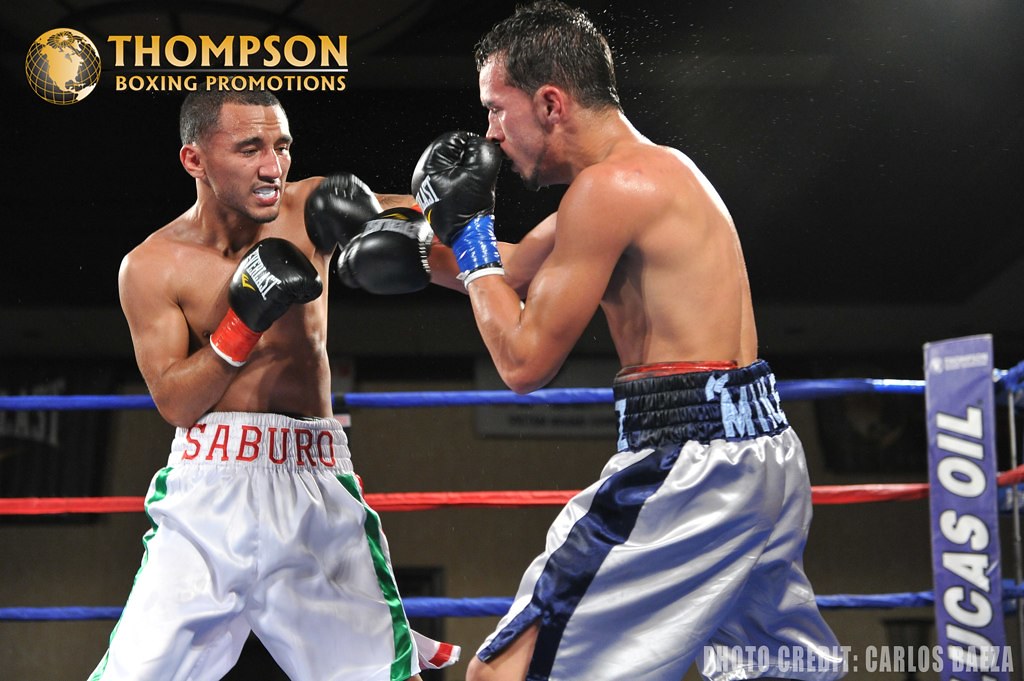This photograph captures an intense moment in an indoor boxing match between two boxers. The boxer on the left, sporting very short dark hair, is clad in white shorts with green stripes and "Saburo" written in red across the waistband. The boxer on the right, identified by short dark hair as well, is wearing light purple shorts accented with black lines. Both athletes, equipped with black boxing gloves, are captured mid-swing, fully engaged in the bout. Surrounding the fighters are the blue and red ropes of the ring. In the top left corner of the image, a golden logo featuring a globe and the text "Thompson Boxing Promotions" stands out against a dark background. Additionally, the bottom right corner of the photograph credits Carlos Baeza as the photographer. Not much can be seen beyond the ring, but to the right, vertically printed blue text reads "UCAS space oil."